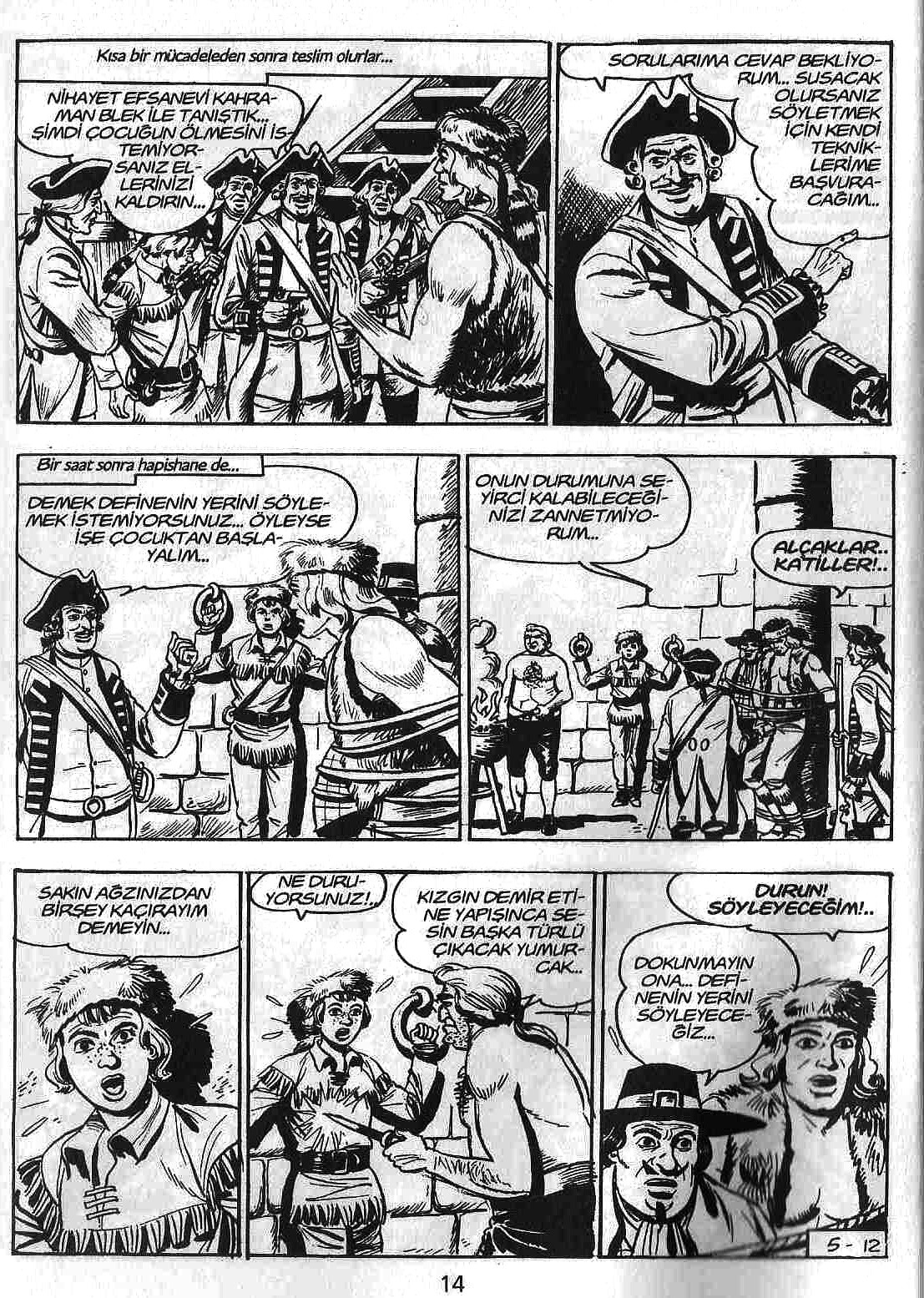This black-and-white comic strip, potentially resembling a newspaper cartoon, is divided into seven panels with discernible yet non-English text. It depicts a dramatic scene, possibly related to pirates or military personnel, capturing several characters. The top row features two panels; the first shows several men in military attire alongside one man with a distinctive fur hat resembling a raccoon or beaver tail, and the second highlights a military man speaking. In the center row, the left panel reveals the fur-hatted man tied to a pillar, with a military figure speaking and another person shackled to a wall, while the adjacent panel showcases both captives with surrounding military men. The bottom row has three panels: the left depicts the fur-hatted man angrily shouting, the center shows an individual approaching the shackled man wielding a knife, and the rightmost panel introduces a character dressed as a pilgrim next to the fur-hatted man. The entire scene culminates on page 14, indicated by the number at the bottom of the page.